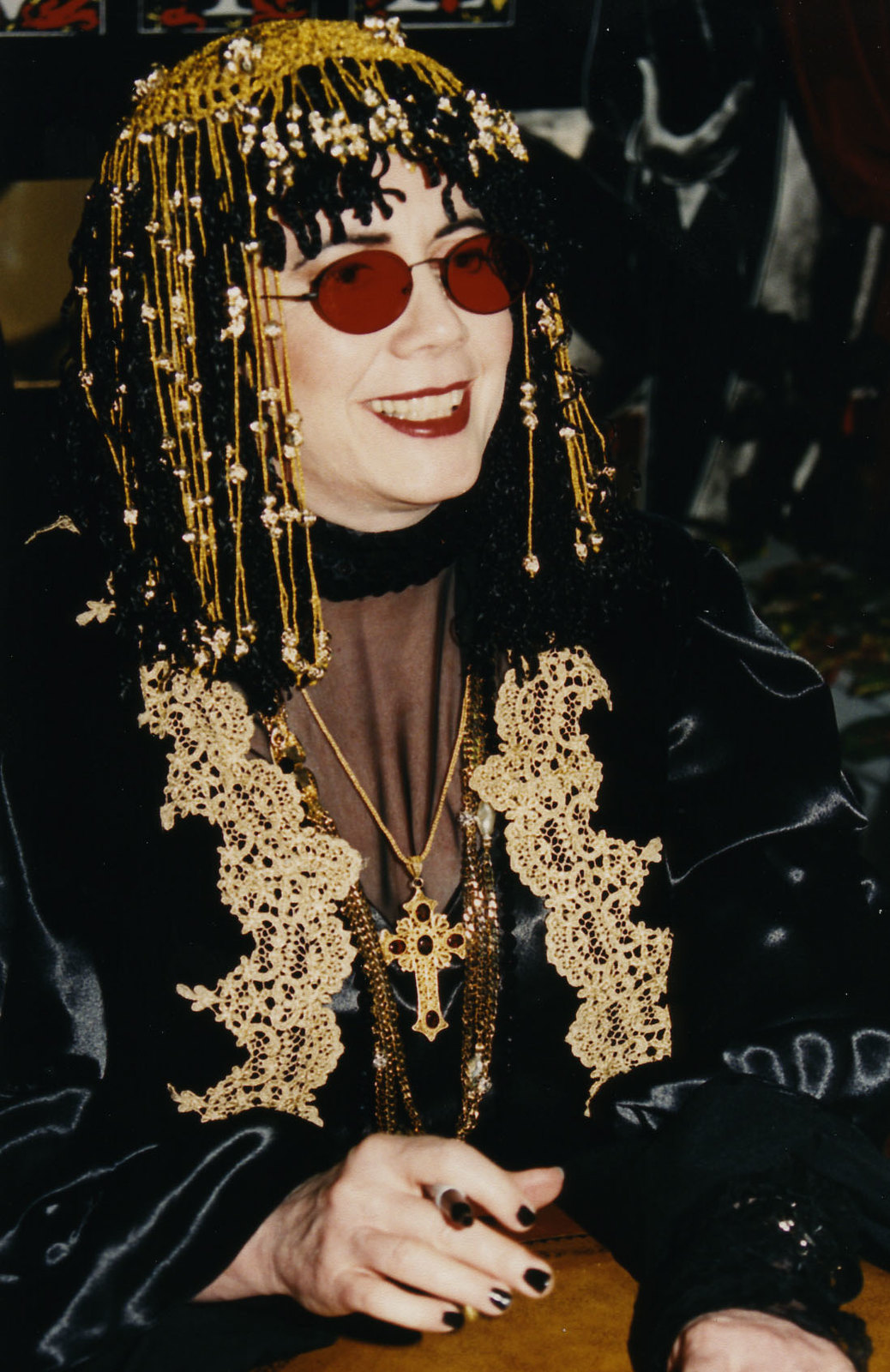In this detailed photograph, a woman occupies almost the entire frame with a confident and radiant presence. She sits indoors against a dark background, possibly signing autographs, and holds a Sharpie marker in her right hand. Her striking accessories include rimless red sunglasses and dark red lipstick that highlights her warm smile. The woman is dressed in a luxurious black satin outfit adorned with gold trim and intricate embroidery, giving her an elegant appearance. Her attire is complemented by several gold chains, the most prominent of which features a large gold cross set with black jewels. Her dark hair is styled in a unique manner, resembling a mix between thin dreads and an Egyptian-inspired headdress with golden lines or beads woven into it. Her nails are painted black, adding to her sophisticated look. Overall, the image captures her poised and stylish demeanor against a simple yet effective backdrop.